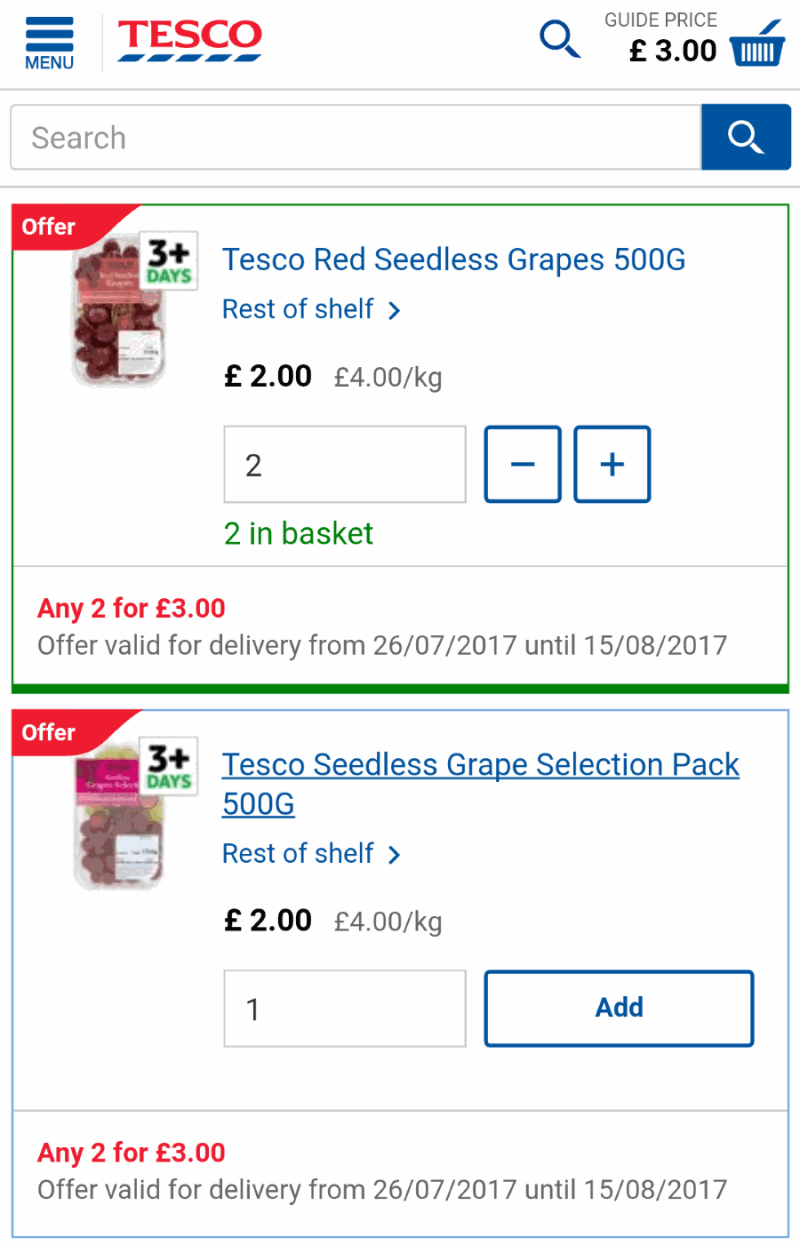This screenshot displays two promotional offers from Tesco. The Tesco logo is prominently featured in uppercase red letters with a fragmented blue line underneath it. In the upper left corner, there is a three-bar menu labeled "Menu." To its right, a microscope icon signifies the search function, followed by a guide price, which is approximately three pounds, and another microscope icon next to a search box.

The first offer showcases an image, slightly fuzzy and small, that seems to depict red grapes. The label indicates "3+ days" for freshness. The official product name is "Tesco Red Seedless Grapes, 500 grams, Rest of Shelf." The price for this item is two pounds, and it is indicated in green that two units are currently in the basket. The offer is valid from July 26, 2017, to August 15, 2017.

The second offer features the "Tesco Seedless Grape Selection Pack, 500 grams," priced at two pounds, which equates to four pounds per kilogram. Presently, only one unit of this item is selected.